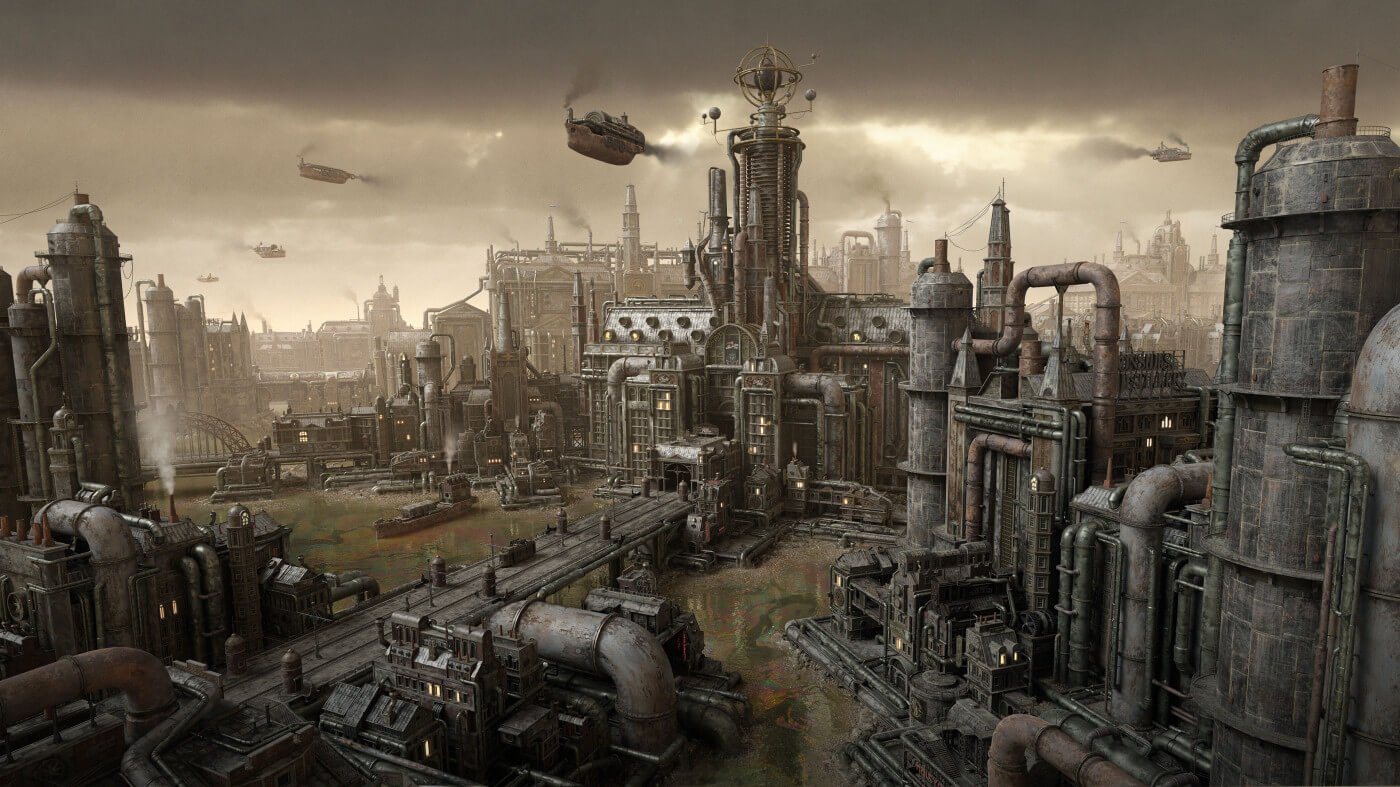A computer-generated depiction of a massive, dystopian industrial factory complex spanning both sides of a smoky, dark gray sky. In the center, a large bridge connects the main factory building to another section, while a polluted river runs beneath it, lending an ominous aura to the scene. The factory, characterized by its old, dark brown and silver hues, is surrounded by numerous towering smokestacks and intricate networks of pipes, contributing to the pervasive haze. The industrial cityscape, built predominantly on water, features flying steampunk-inspired ships, emanating steam and smoke. One ship is prominently displayed in the middle of the image, closer than the others. Despite a few dimly lit windows, the majority of the factory's structures are devoid of light, amplifying the grim, futuristic atmosphere.